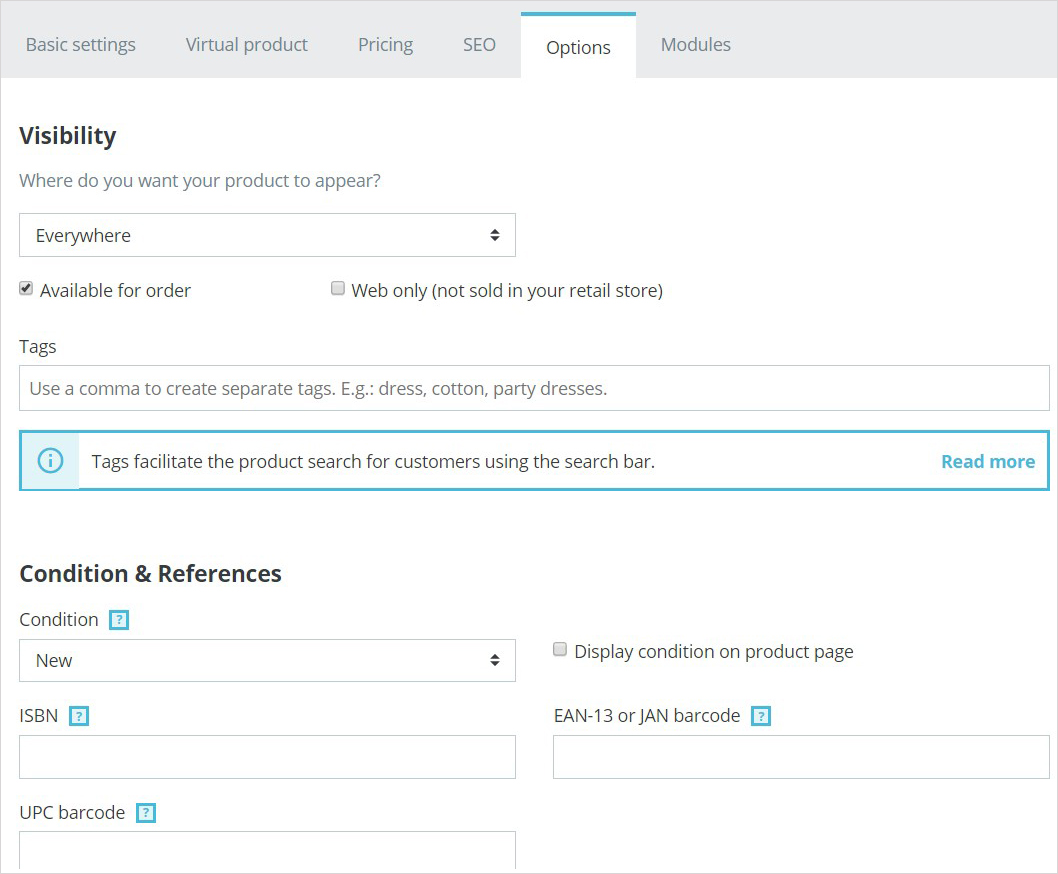In this screenshot of an application's settings section, the interface is organized for easy navigation. At the top, a gray bar contains various menu options labeled "Basic Settings," "Virtual Product," "Pricing," "SEO," "Options," and "Modules." The user has selected the "Options" menu, which is highlighted in white.

Underneath this menu, there is a white screen with text in black font. The first section, labeled "Visibility," poses the question, "Where do you want your product to appear?" A dropdown menu below this question shows that the user has chosen the option "Everywhere." 

Further down, the label "Available for Order" is next to a selected checkbox, indicating that the product is available for order. Another option reads "Web only (not sold in your retail store)," but this option remains unselected.

The section titled "Tags" features a field where users can input tags. The placeholder text provides examples of how to use commas to separate tags, such as "dress," "cotton," and "party dresses." Below this input field is an outlined blue rectangle with white in the center explaining that "Tags facilitate product search for customers using the search bar." This note includes a "Read more" link for additional information.

Lastly, the section labeled "Conditions and References" is also present in black font, but no specific details are filled in.